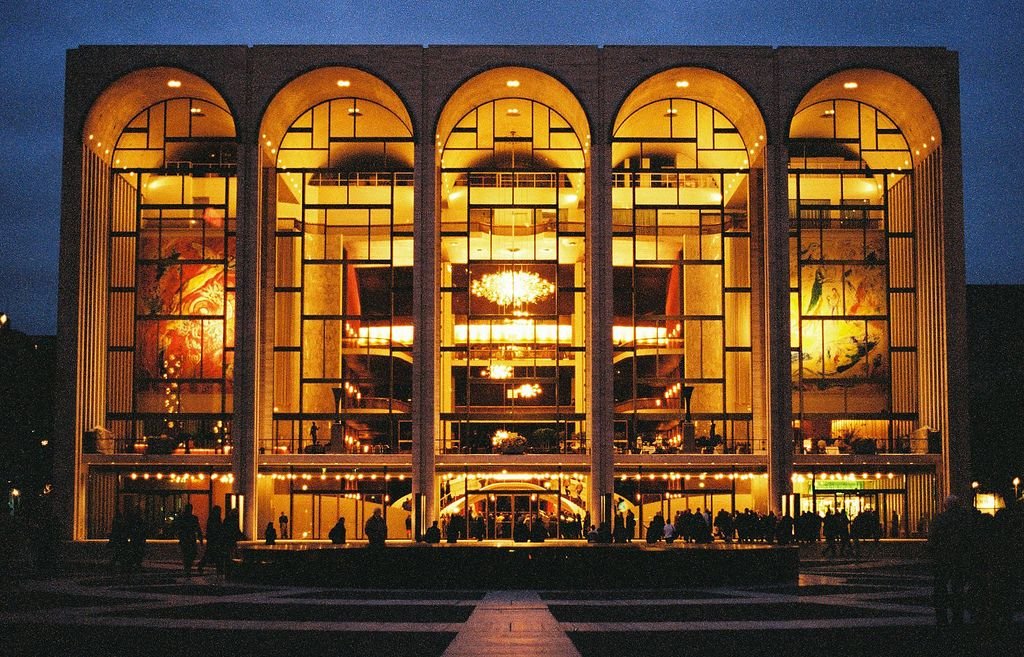The image captures a night-time view of the Metropolitan Opera building in New York. The rectangular structure prominently features five tall, arch-shaped sections on its front, which resemble towering cylindrical forms. Each of these arches has a framed outline and large glass windows, allowing a clear view into the brightly illuminated interior. The lighting inside is a warm, bright yellow, creating a striking contrast against the deep blue night sky. At ground level, multiple doors are visible, flanked by people entering or silhouetted against the building's light. Inside, the details are crisp; paintings adorn the far right and left walls, and an ornate chandelier hangs from the ceiling. The building’s design includes window patterns reminiscent of Mondrian's black grid lines, and the overall atmosphere is one of grandeur and cultural significance.